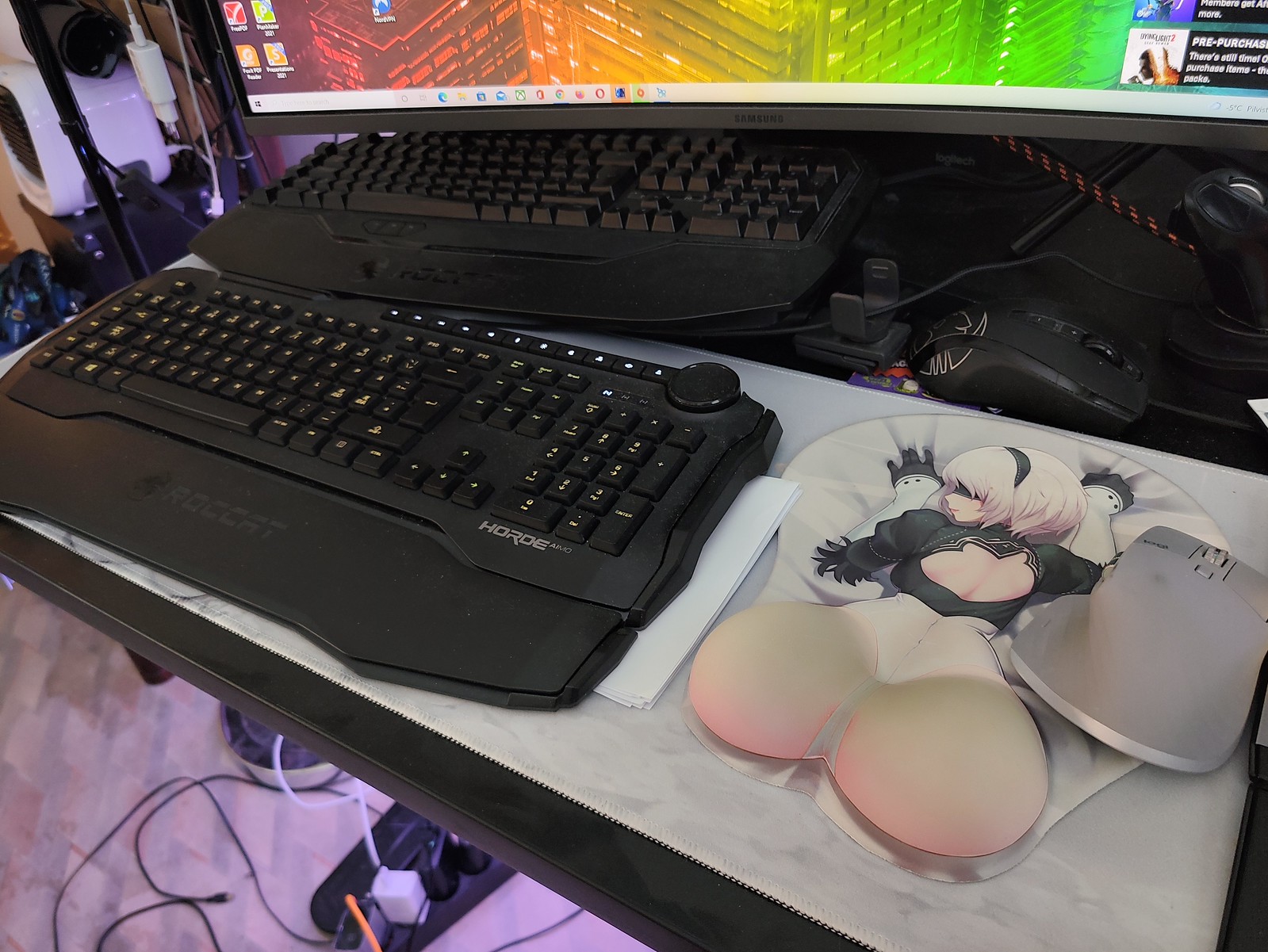This photo showcases an elaborate desk setup featuring a unique pullout drawer. On top of the white main desk sits a large monitor with a windowed, rainbow-colored background, adorned with icons on the left and images on the right. The pullout portion of the desk holds two black keyboards; the front keyboard has a wrist rest extension. To the side of the keyboards lies a mouse pad depicting a Japanese anime character—a woman with a black headband, blonde hair, gloves, and a bare bottom, with her back turned and arms outstretched. A contemporary, light gray mouse is positioned atop the mouse pad. The surrounding area is cluttered with various cables, a power strip with multiple plugs, and a white alarm clock with a black face. The purple-hued floor beneath the desk features a visible power supply unit with numerous cables plugged into it.